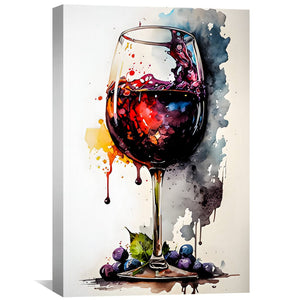The image showcases a vibrant watercolor painting centered around a wine glass, brimming with a kaleidoscope of colors including purples, oranges, reds, and blues. The glass seems to be capturing a dynamic moment, as if wine is still being poured, creating splashes and splatters that decorate the canvas around it. At the base of the wine glass, an assortment of fruits—grapes and blueberries—along with a green leaf, add to the detail and charm of the scene, with additional splatters underneath enhancing the sense of movement. The background is a medley of watercolor splatters featuring shades of brown, light gray, blue, black, and streaks of yellow and red, creating a rich, textured backdrop that complements the vivid composition of the glass and fruits.